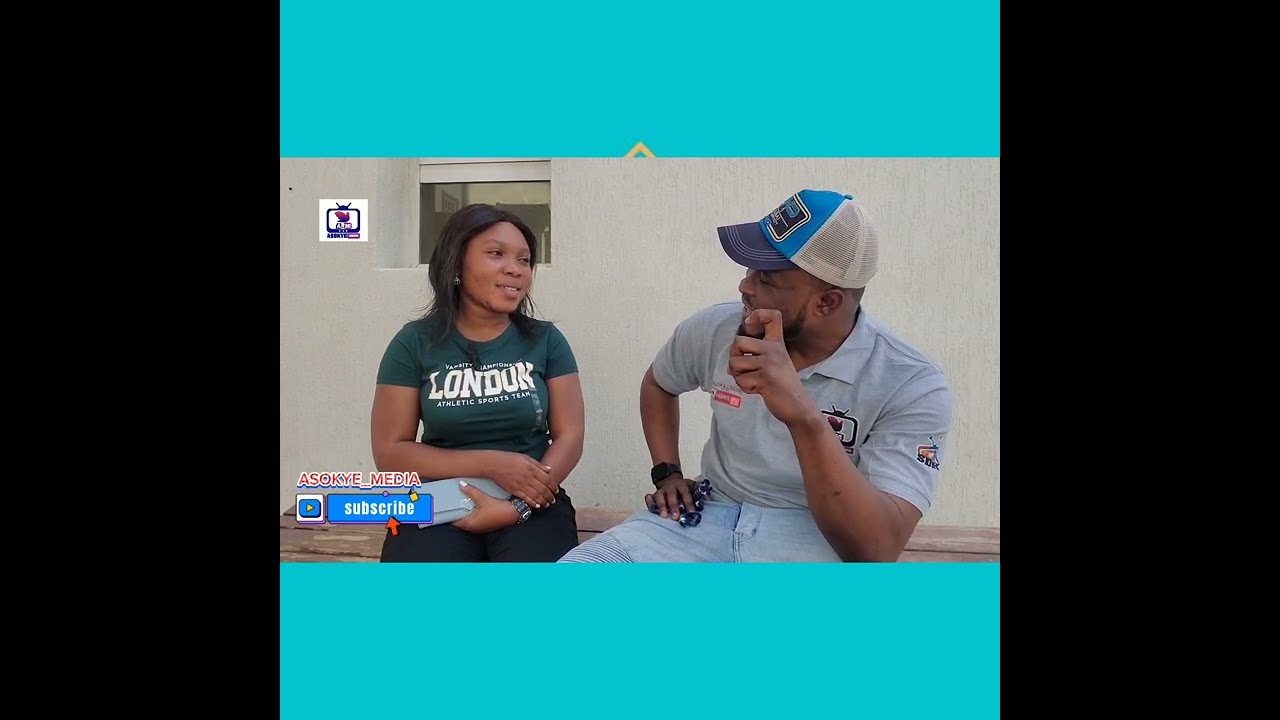The image appears to be a still from a video, potentially a YouTube clip or social media content, featuring two people engaged in a conversation while sitting on a wooden bench against a beige wall. On the left side of the image, there is a woman with dark brown skin and shoulder-length black hair. She is dressed in a green t-shirt that prominently displays the text "London" and below it in smaller letters, "Athletic Sports Team." She's wearing black pants and smiles as she looks at the man beside her. On the right, the man, who also has dark skin and a beard, is wearing a gray polo shirt paired with light blue jeans and a baseball cap that has a light blue front, dark blue brim, and a white back. His left arm supports his head as he converses with the woman. Additionally, he holds a handbag. In the bottom left corner of the image, the text "ASOKYE Media" is visible along with a logo encouraging viewers to subscribe.